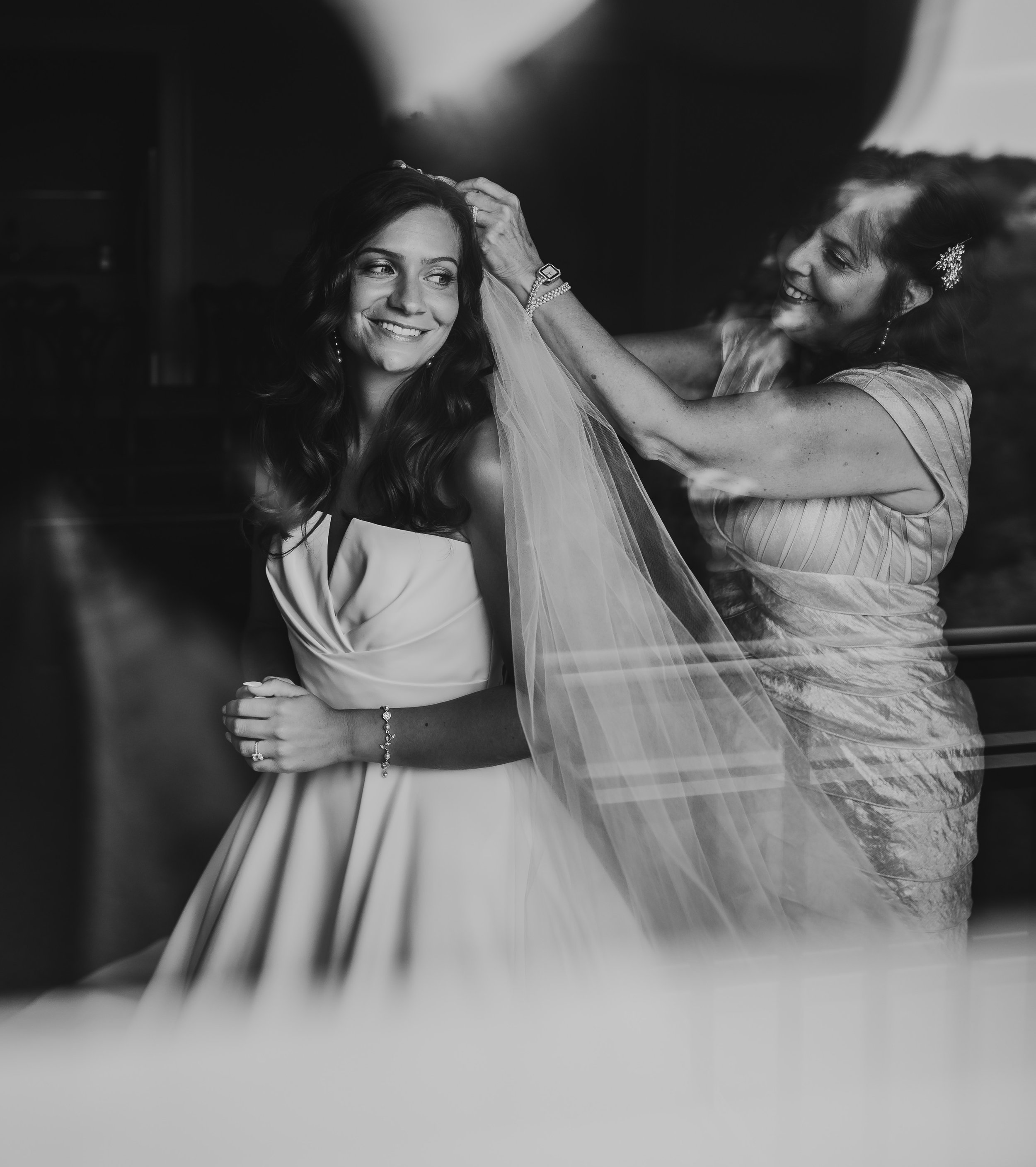This black and white photograph, likely taken by a professional photographer, captures an intimate and joyful moment as a bride prepares for her wedding day. The focus is on two women, the bride, and an older woman who is presumably her mother. The bride, standing in a beautifully detailed white wedding dress, looks back with a radiant smile at the woman assisting her. Her hair is elegantly curled, adorned with a veil being carefully adjusted. She wears tasteful jewelry, including a bracelet on her left arm and earrings, enhancing her classic bridal look. The older woman, also smiling warmly, is dressed in a stylish, textured dress and accessorized with a bracelet, a watch, and long earrings. Her hair, which features a notable brooch, is slightly grayed, adding to the timeless quality of the scene. The background is softly blurred, placing prominent emphasis on the touching interaction between the bride and her mother, encapsulating their shared excitement and affection amidst the pre-wedding preparations.